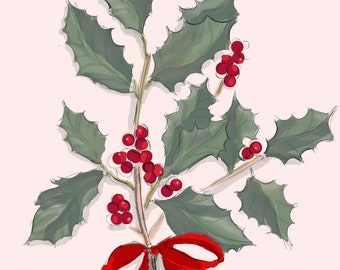This image is a detailed illustration of a holly bush branch, vividly depicting the greenery and festive elements associated with it. The holly leaves are depicted in a subdued, almost olive green, with pointed jagged edges, rendered in a brushed or watercolor style. There are two branches in the image, which are tied together at the base with a red ribbon tied in a bow. Among the green leaves, clusters of 20 red berries are scattered, with many berries concentrated in the middle of the branch and some extending towards the edges. The entire composition is set against a plain white or pastel pink background, enhancing the simplicity and elegance of the watercolor depiction.